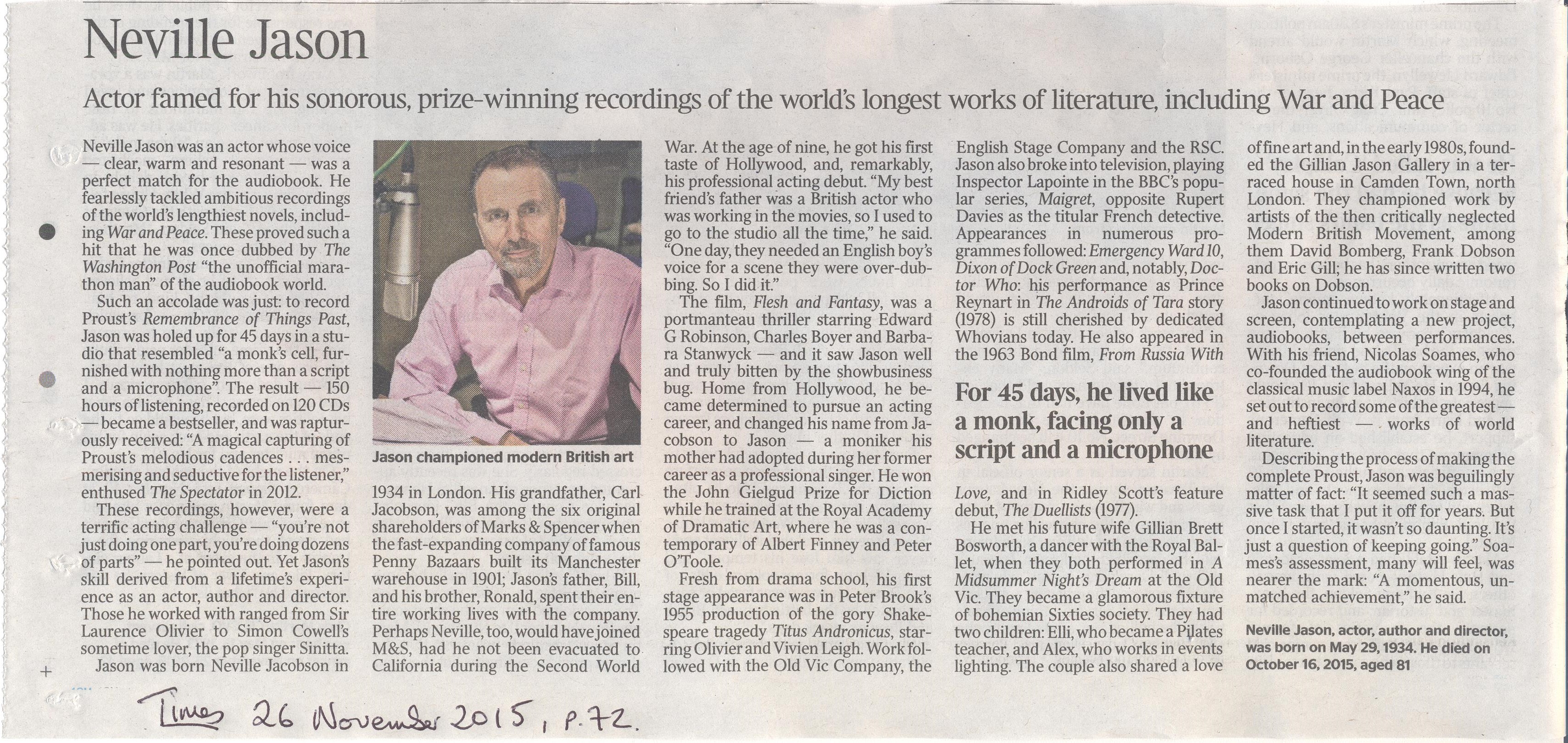The image features a meticulously cut-out newspaper article titled "Neville Jason" in the upper left-hand corner. Below the title, the text describes him as an actor celebrated for his award-winning recordings of the world's longest literary works, including "War and Peace." The article has been neatly excised from its original context, evidenced by visible scissor marks along the top edge and slightly jagged sides, indicative of its newspaper origin.

Prominently displayed in the article is a photograph of Jason Chipperman, who is depicted wearing a pink button-down shirt. The accompanying subtext highlights his advocacy for modern British art. Chipperman appears to be seated in a nostalgic interview setting, complete with an old-fashioned hanging microphone, suggesting a moment from a past era of broadcasting.

Handwritten annotations on the lower left corner of the article read "Tuesday, times 26, November, 2015," followed by "P72," suggesting a specific date and page for the article. The narrative of the article delves into the life of Neville Jason, focusing on a remarkable 45-day period during which he lived ascetically, engaging solely with a script and a microphone. The description underscores his dedicated, almost monastic approach to his craft, reflecting on his life and achievements in greater detail.